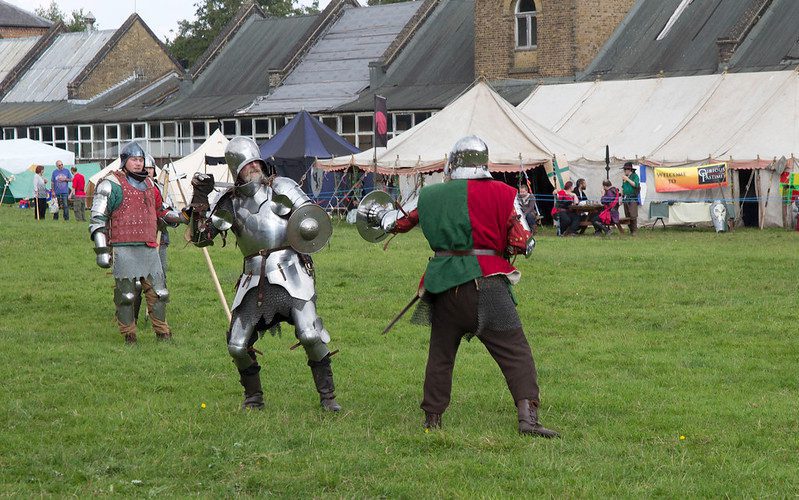In the foreground of the image, two men are engaged in a medieval sword fight re-enactment on a green grassy field. The man on the left is clad in full silver armor with an oversized helmet, brown leather boots, and a small buckler shield held out in his left hand. His right hand holds a sword casually draped over his shoulder. He appears to have a gray beard. His opponent, positioned on the right with his back facing the camera, is wearing a two-toned cotton shirt—green on the left and red on the right—along with brown pants, black boots, a leather belt, and a silver helmet. He also holds a similar small buckler shield in his left hand and appears to have chain mail underneath his shirt. 

In the background, there's a noticeable setup of tents, one of which is black while the rest are white, arranged along a green field. Some people are standing around these tents, mingling and dressed either in modern clothes or medieval costumes. Additionally, there is a brown-bricked building with windows and a triangular roof. To the left middle behind the fighting pair, another man in medieval attire, featuring a red vest, silver gauntlets, and a helmet, stands observing the duel. This scene vividly re-creates a medieval festival or event with details that suggest a historical re-enactment ambiance.